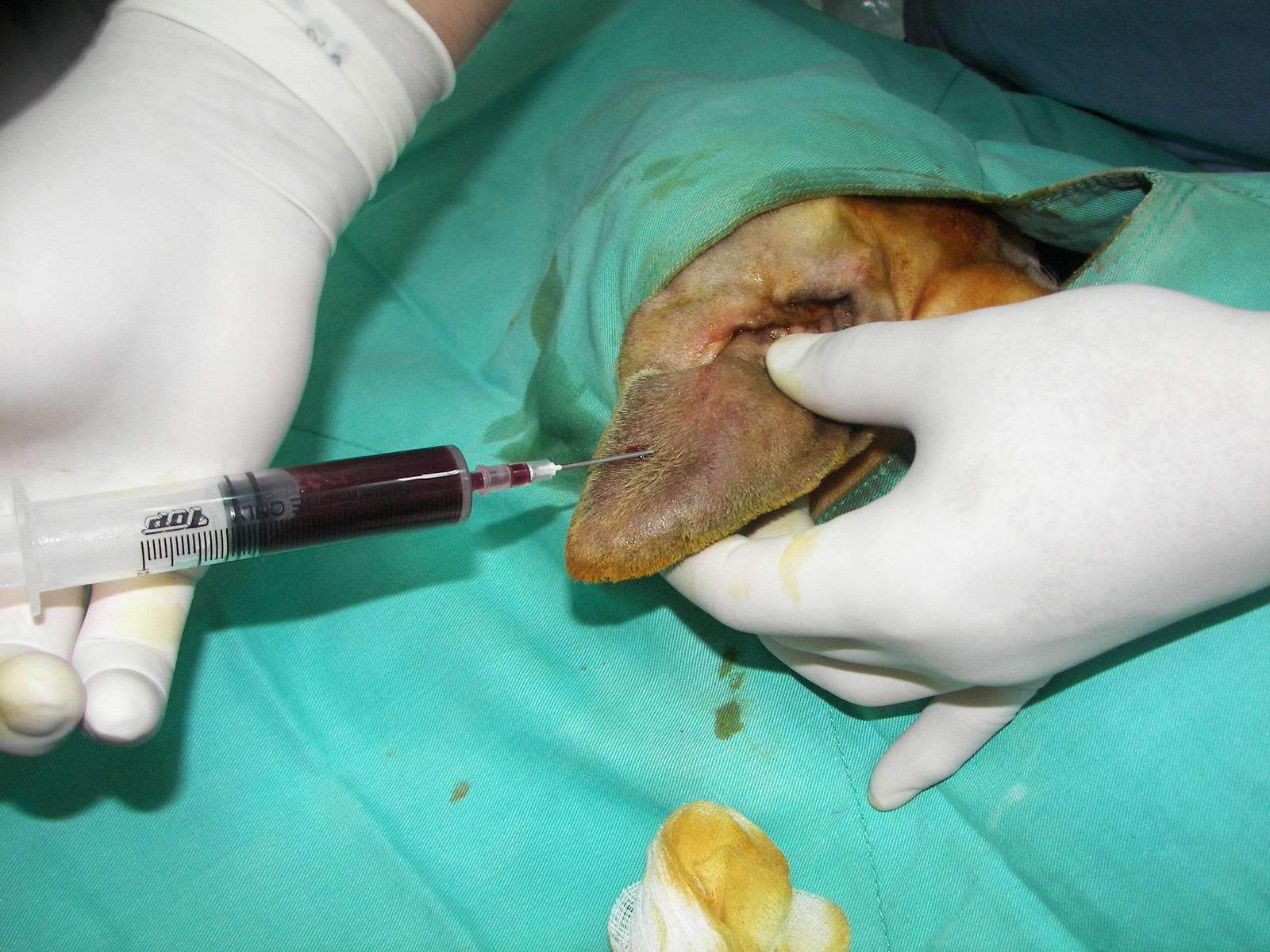The photograph captures a close-up of a veterinary procedure on an animal, likely a dog. The image centers on a green surgical drape with a hole through which a portion of the animal's body, probably an ear, is visible. The ear, covered in short, blondish fur, is being handled by a person wearing white latex gloves. The vet is injecting a syringe filled with a dark, possibly maroon or black serum into the ear. Surrounding the injection site is a small blot of iodine, indicating a sterile area. In the bottom center of the photo, there's a piece of gauze or cotton ball stained with a yellowish, oily substance, possibly from the procedure. The overall focus is on the detailed precision of the veterinary work being conducted.